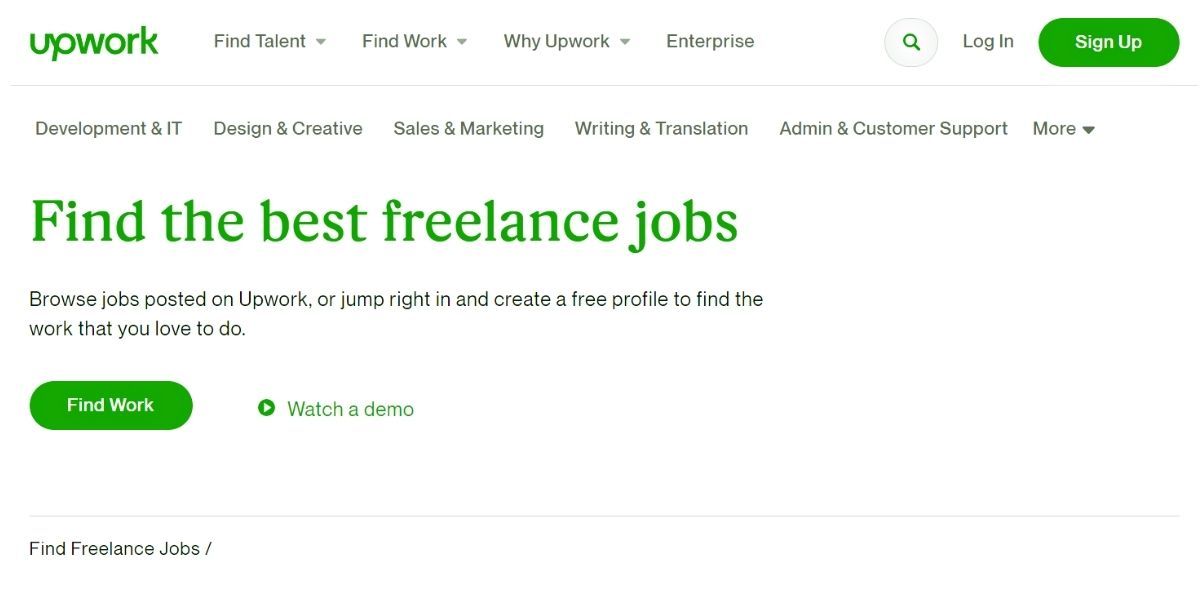Screenshot of the Upwork website homepage. The top left corner features the green Upwork logo with a stylized "P." The top navigation menu includes the following buttons: "Find Talent" (drop-down), "Find Work" (drop-down), "Why Upwork" (drop-down), "Enterprise," a green search icon, a login button, and a green pill-shaped sign-up button. Below the navigation menu is a secondary horizontal menu with categories separated by vertical lines: "Development & IT," "Design & Creative," "Sales & Marketing," "Writing & Translation," "Admin & Customer Support," and more (drop-down). Prominently displayed below this menu is a headline in large green text that reads, "Find the Best Freelance Jobs." Underneath, a subtext invites visitors, "Browse jobs posted on Upwork or jump right in and create a free profile to find the work that you love to do."